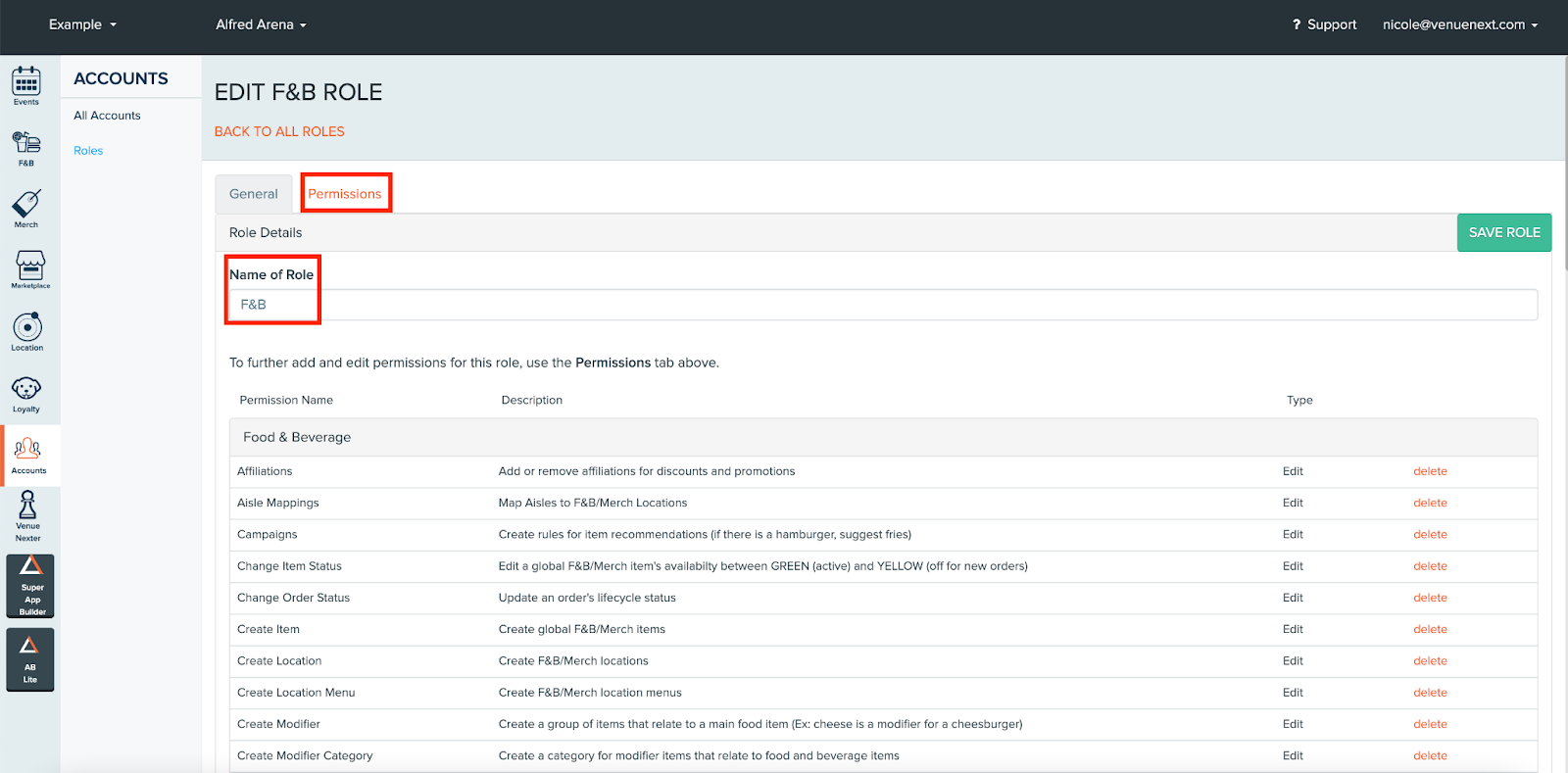This image is a detailed screenshot of a backend dashboard for a website or software. At the very top, a dark gray navigation bar stretches across the width of the interface. The left side of this bar features dropdown buttons labeled "Example" and "Alfred Arena." On the right side, there are a question mark icon, a "Support" link, and a dropdown menu for user account settings, which displays "Nicole at VenueNext.com" when expanded.

On the left side of the screen, a vertical sidebar presents a series of icons with small labels underneath. This sidebar is primarily light gray, containing eight gray buttons, followed by two dark gray buttons at the bottom of the list.

Adjacent to this sidebar is another vertical gray section titled "Accounts." Below this header, there are two subsections: "All Accounts" and, highlighted in blue, "Roles."

The central part of the screen prominently showcases the editing interface for roles. At the top left, the section is titled "Edit F&B Role." Just beneath this, an orange link states "Back to All Roles." The interface below this is divided into two gray tabs labeled "General" and "Permissions." The "Permissions" tab is currently active, indicated by a red box that surrounds it.